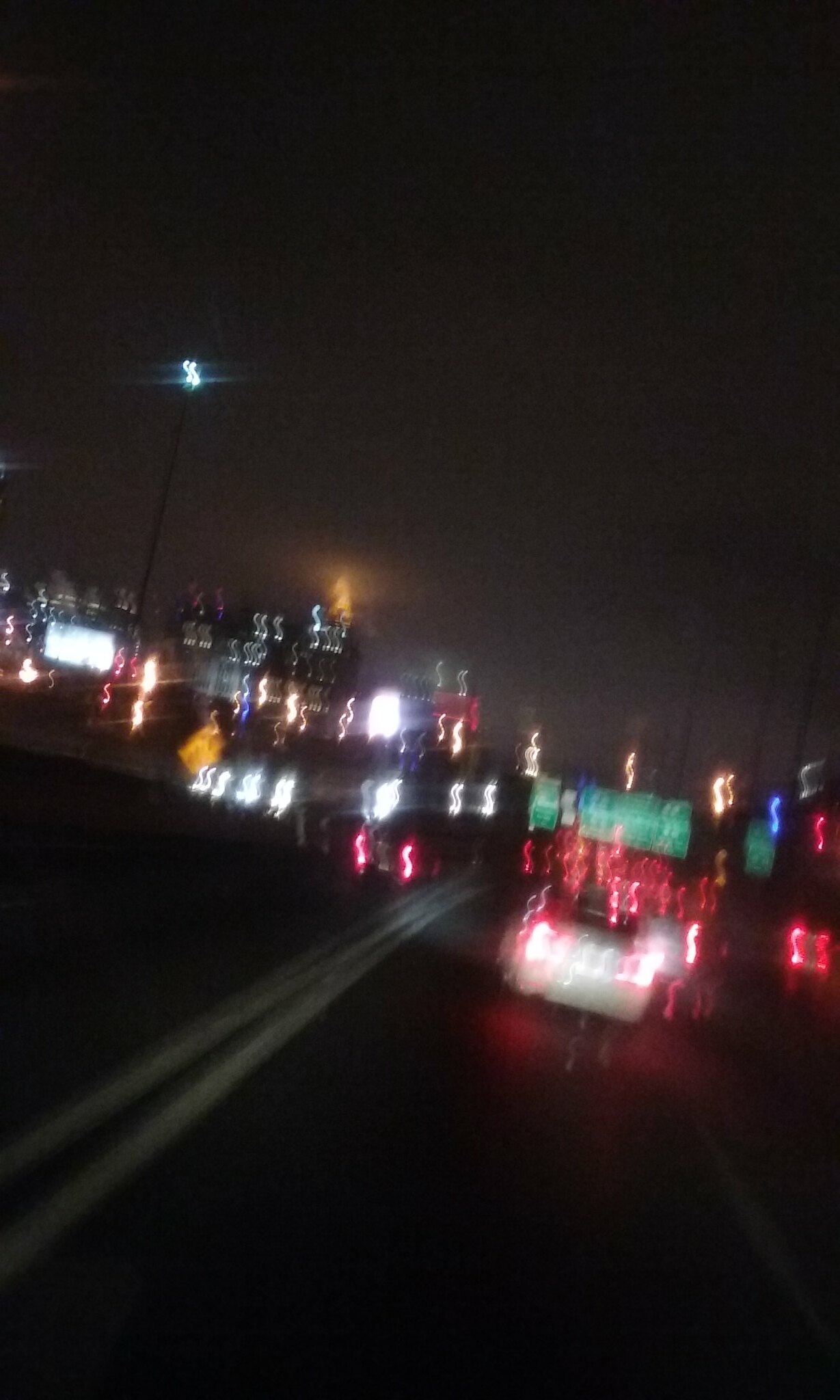This vertically oriented, nighttime photograph, captured through the windshield of a car, offers a blurred, surreal glimpse of urban life. Dominated by shades of black and gray, the image is punctuated by vibrant streaks of color from city lights, buildings, and vehicle headlights and taillights. Along the center, two yellow lines stretch diagonally from the lower left corner, guiding the eye through the frame. Amidst the ambient luminescence, green street signs can be seen hovering in the central part of the photograph, adding to the metropolitan feel. A streetlight peeks through gaps between the towering silhouettes of buildings. The top portion of the image is enveloped in darkness, creating a stark contrast with the scattered, multicolored lights that define the cityscape below. Of particular prominence is a slightly larger car ahead of the viewer, distinguishable amid the abstract forms. The overall impression is one of motion and anonymity, an evocative capture of a fleeting moment on the city roads.